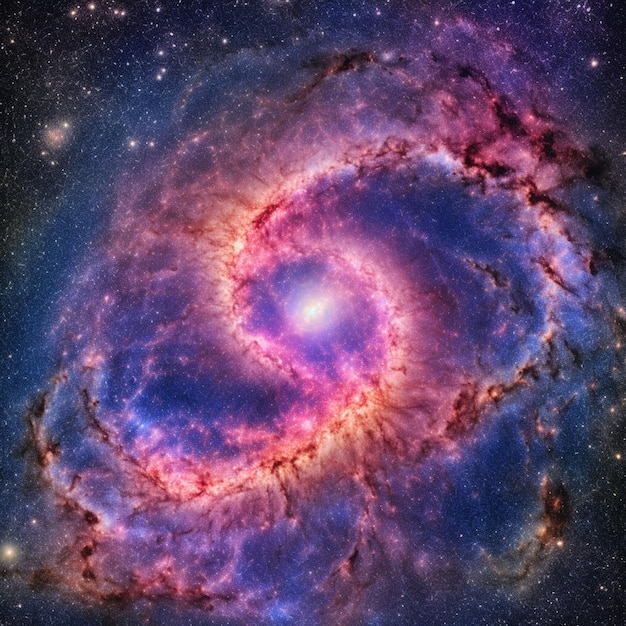The image depicts a captivating, possibly computer-generated or AI-generated, representation of a spiral galaxy. It features a multitude of stars scattered around the outer edges against a backdrop of deep black and blue. At the center, there's a radiant, small ball of bright white light, surrounded by intricate swirls of pink, purple, and occasional dark red hues. This central light could be interpreted as a sun or perhaps the core of a nebula. The swirling arms of the galaxy extend outward in cosmic spirals, lending a dynamic, expansive feel to the scene. Various vibrant colors—ranging from oranges to pinks—mix harmoniously, enhancing the otherworldly aesthetic of this deep space depiction.